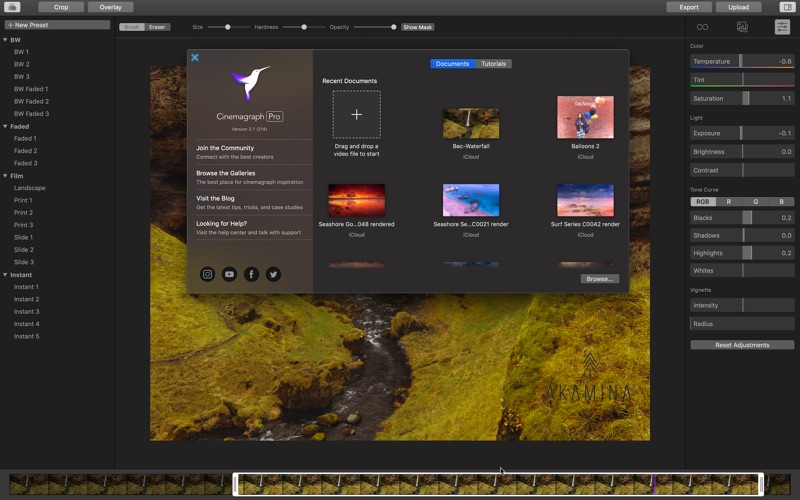**Descriptive Caption:**

This screenshot captures the interface of the Cinemagraph Pro application, featuring a modern dark theme designed for video editing. At the center of the screen, a pop-up window prominently displays the Cinemagraph Pro logo along with the version number 2.7.4.244. This window includes sections for community engagement, navigating galleries, visiting the blog, and seeking assistance, demonstrating the app's support features.

Adjacent to the pop-up, thumbnail previews of recent projects—including titles like "Bee Waterfall," "Balloons 2," "Seashore Go 084 render," "Seashore C0021 render," and "Surf Series C0004 render"—provide quick access to ongoing work. The left sidebar is equipped with a selection of filters, including BW (black and white) and Instant, alongside the option to create new custom presets, enhancing creative possibilities.

Above the central editing workspace, users can find critical adjustment tools for brush size, hardness, opacity, and toggling mask views, facilitating detailed edits. The right sidebar offers comprehensive color adjustment controls, covering essentials such as temperature, tint, saturation, exposure, brightness, and contrast, emphasizing the app's robust color correction capabilities.

At the top right corner, buttons for exporting and uploading streamline the workflow process. The background reveals the primary editing area, showcasing a landscape scene featuring a serene river winding through grassy terrain. Finally, a timeline at the bottom of the screen displays video frames as thumbnails, enabling precise editing.

Overall, Cinemagraph Pro's interface is thoughtfully designed to be user-friendly while providing powerful video editing and color correction tools, catering to both novice and experienced users.